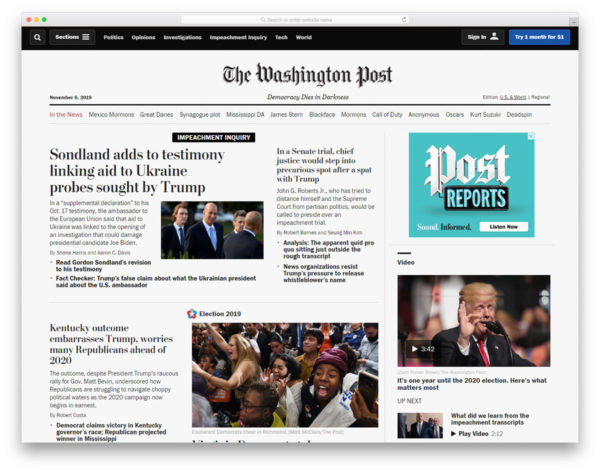This image is a screenshot of a webpage displayed on a Mac computer, indicated by the characteristic red, yellow, and green control buttons in the top-left corner. At the top center of the screen, there is a white search bar. Dominating the mostly white background of the webpage is a thin black bar across the top, which features various navigation buttons labeled: "Search," "Sections," "Politics," "Opinions," "Investigations," "Impeachment Inquiry," "Tech," and "World," all in white text. On the right end of this black banner, there's a black "Sign In" button and a blue "Try one month for $1" button in white text.

Centered in the middle of the webpage, prominently displayed, is "The Washington Post" in bold. Below this, in smaller text, the date "November 6, 2019" is positioned on the left, and the paper's motto, "Democracy Dies in Darkness," is centered beneath the title. The rest of the page features various articles and accompanying images. 

The primary headline, centrally located, reads: "Sondland adds to testimony linking aid to Ukraine probes sought by Trump," alongside a photo of men in suits. Another significant article below it, titled "Kentucky Outcome Embarrasses Trump, Worries Many Republicans Ahead of 2020," occupies a prominent position on the page. 

In the bottom right corner of the webpage, there's an image of Trump with a headline reading "Video: It's one year until the 2020 elections. Here's what matters most." A teal square labeled "Post Reports" on the middle right side of the page serves as an advertisement with the slogan "Sound informed."

Overall, this detailed webpage from The Washington Post includes a variety of features intended to provide comprehensive news coverage and facilitate user navigation.